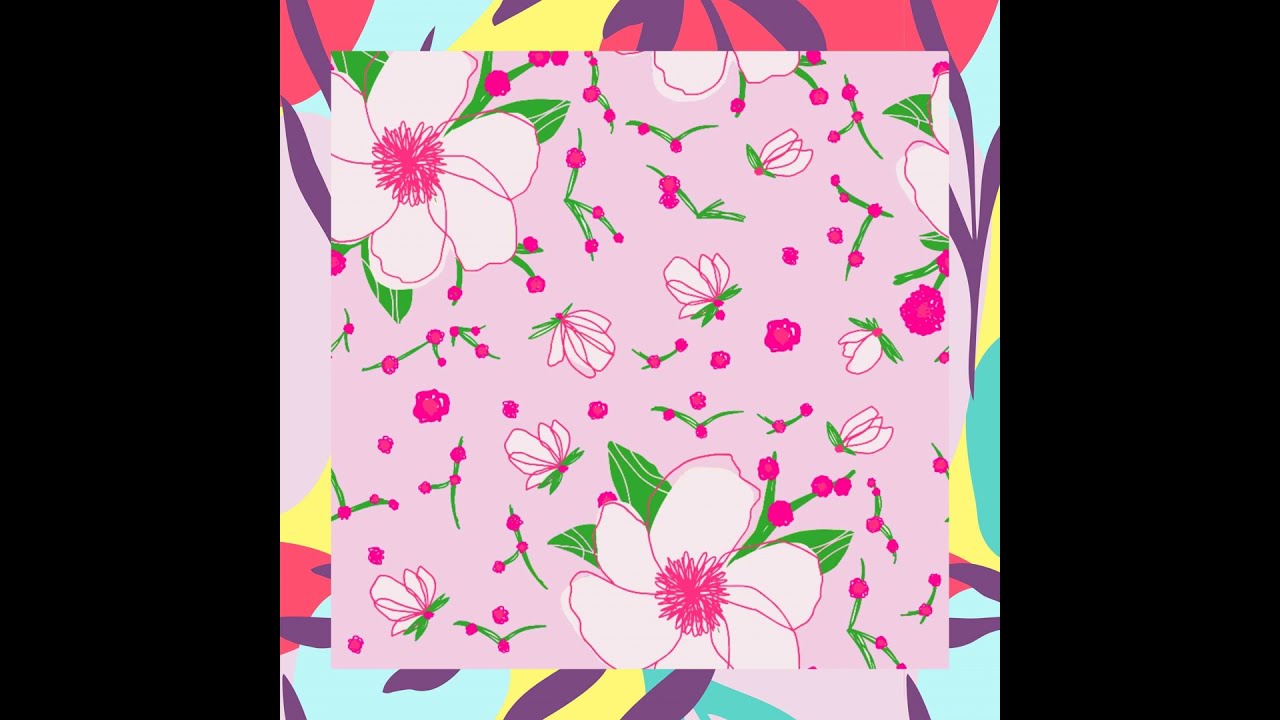This image showcases a digital drawing that resembles a collage-style piece of wallpaper art. Central to the composition is a large square adorned with a floral pattern. The background of this central square is a pastel pink color, featuring an array of white flowers with some having pink sprinkles at their centers. These predominant flowers are accompanied by clusters of smaller flowers, some drawn in a stylized, sketchy manner with pink outlines. Interspersed among the flowers are pastel-colored elements in blue, purple, and yellow, giving the design a soft, dreamy quality. The flowers seem to float over a layer of another floral image in contrasting colors, creating a layered effect.

Surrounding this central floral square is a border that looks like an abstract collage with vibrant yet soft hues of light purple, dark purple, red, yellow, and light blue. This border complements the central floral motif while adding a touch of artistic abstraction, making the overall image appear both feminine and intricate. The varied colors and the stylized design render it reminiscent of decorative art you might find on a girl's school folder or similar stationery.